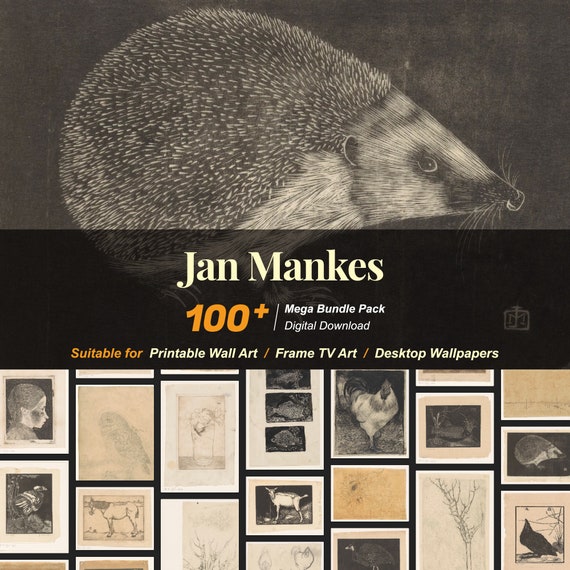This image serves as a promotional advertisement for Jan Mankes' "100 Plus Mega Bundle Pack Digital Downloads." Dominating the upper half, a dark background features a monochromatic illustration of a porcupine, showcasing its distinctive quills, triangular face, visible eye, ear, and dark nose. Across the middle, a black horizontal strip highlights key promotional text: "Jan Mankes" in white lettering, and directly below, "100 Plus Mega Bundle Pack Digital Download" with "100 Plus" emphasized in orange. A secondary line reads in orange and white that the pack is "suitable for printable wall art, frame TV art, desktop wallpapers."

The lower half of the image displays a grid of 10-12 muted illustrations, predominantly featuring animals such as a rooster, goat, and another porcupine, along with human faces, birds, trees, and other natural themes. These artworks maintain a consistent color scheme of muted oranges and browns, presented in black frames. This detailed composition effectively showcases the variety and thematic cohesion of Jan Mankes' artistic offerings, focusing on promoting the versatility and aesthetic appeal of her digital download collection.